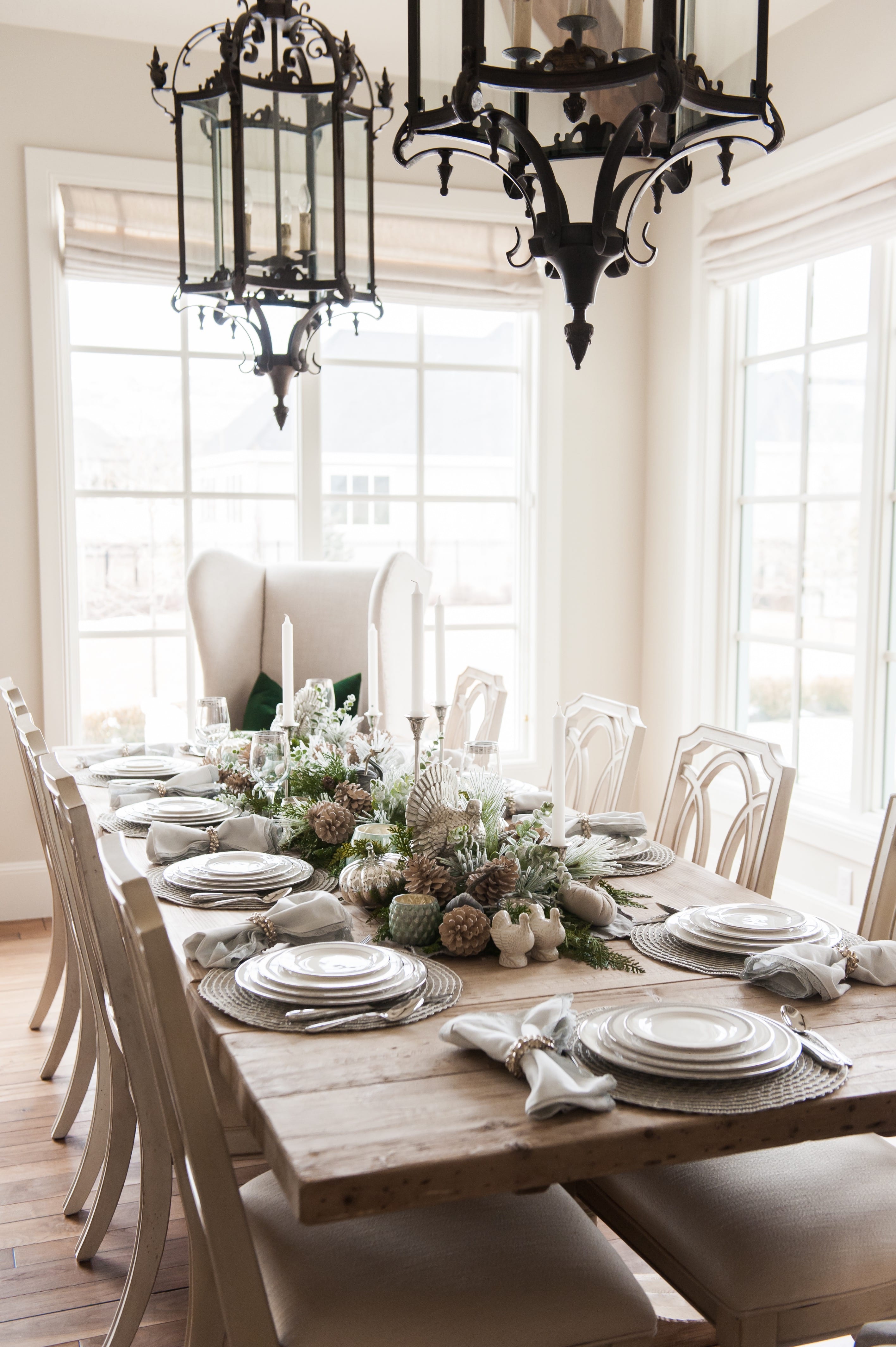The photo captures an elegantly decorated dining room bathed in natural light from large, brightly lit windows on the right and back walls. The rectangular dining table, made of light pine wood, is set formally with woven natural-colored round placemats at each of its eight seats. Four white plates are stacked at each setting, accompanied by elegantly wrapped gray napkins and silver utensils. A centerpiece arrangement of various florals, pinecones, decorative balls, small birds, and white candles, including long stick candles, runs down the center of the table, enhancing the room's romantic and fancy ambiance. The seating comprises basic white chairs, with a distinctive, more luxurious fabric armchair at the table's head, adding a touch of grandeur. The high ceilings feature two ornate black iron chandeliers that complement the overall sophisticated decor of the space.